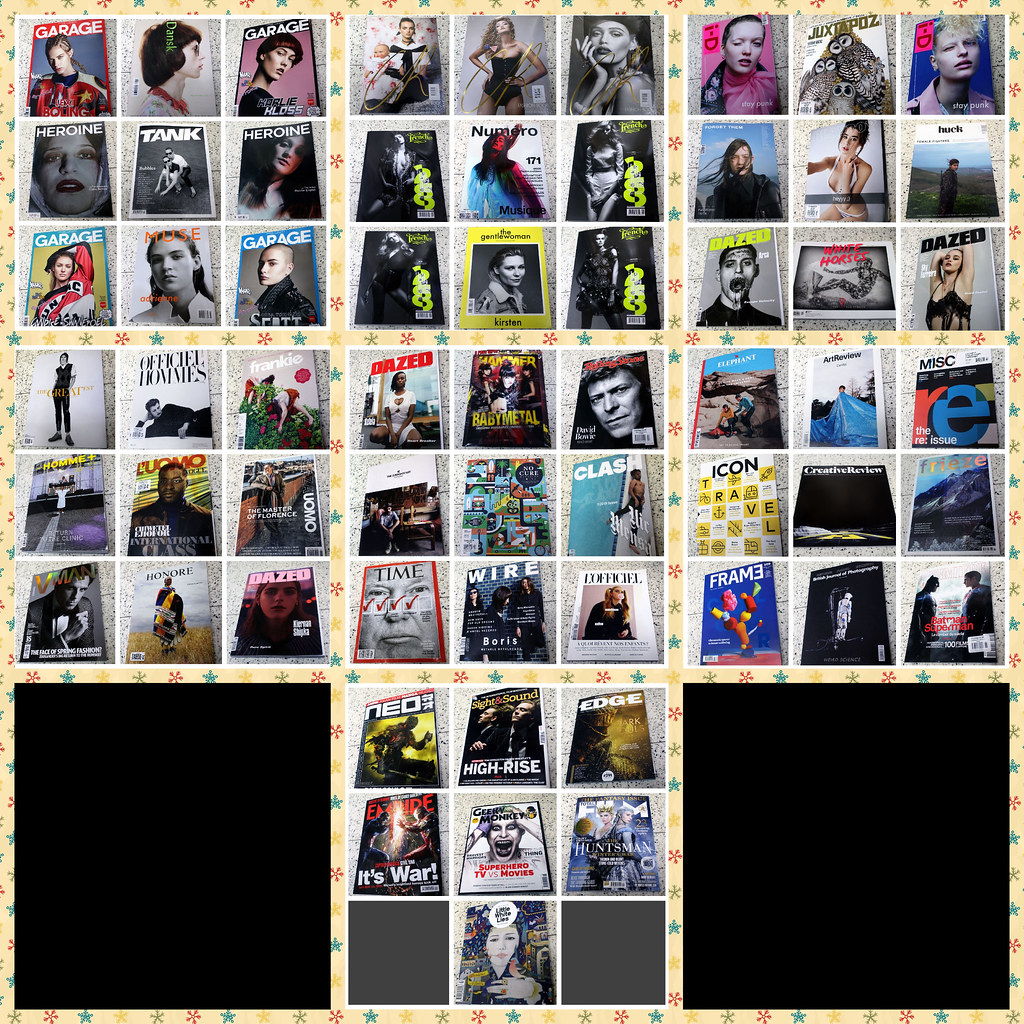The image is a detailed photograph showing seven polaroids arranged in a grid on a patterned surface. The backdrop is a light yellow decorated with various colored stars—blue, red, and green—that evoke the feel of wrapping paper or a festive design. Each polaroid is subdivided into a grid of three by three, forming a collection of nine smaller images within each polaroid. These smaller images appear to be overhead shots of different magazine covers, focusing on culture or music themes. Featured magazine titles include Garage, Muse, Dazed, Empire, Edge, Tank, Heroin, Official Alms, Time, The Wire, and L'Officiel. Intriguingly, out of the seven polaroids, six display sets of nine magazine covers, one shows only seven covers, and two sections are just black, adding an element of curiosity to the composition. The overall arrangement suggests an artistic or visual display, potentially aiming to showcase a variety of magazine aesthetics.